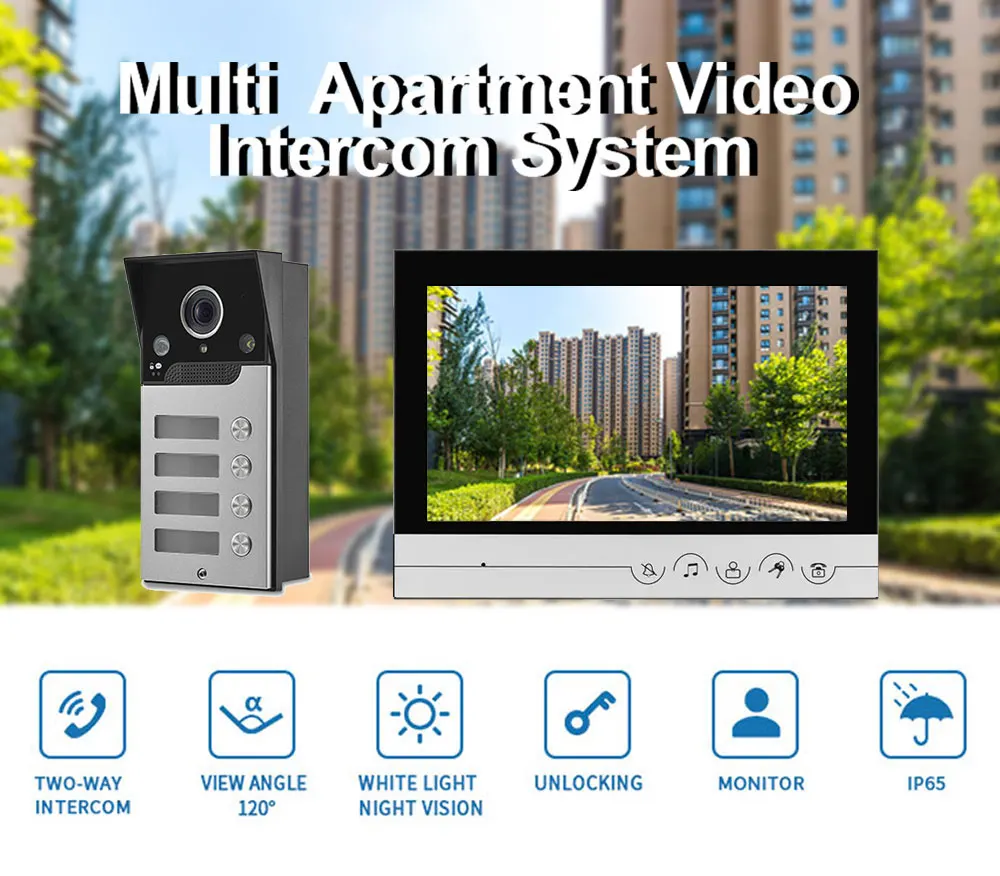The image is an advertisement for a multi-apartment video intercom system, prominently displaying two primary components: a camera entry device and an indoor monitoring screen. In the background, there are several tall, beige and brown high-rise apartment buildings, with a green park-like scene and a road running through it. The foreground features the intercom system; on the left is a black and silver call box with four buttons and a camera, suggesting it can handle up to four apartments. On the right is the indoor monitor with a black bezel and a stainless steel bottom interface, allowing residents to see and interact with visitors. At the bottom of the advertisement, blue text outlines the product features: two-way intercom, 120-degree viewing angle, white light night vision, door unlocking capability, monitoring function, and an IP65 rating, which indicates strong protection against dust and water. The title at the top of the image reads "Multi-Apartment Video Intercom System."